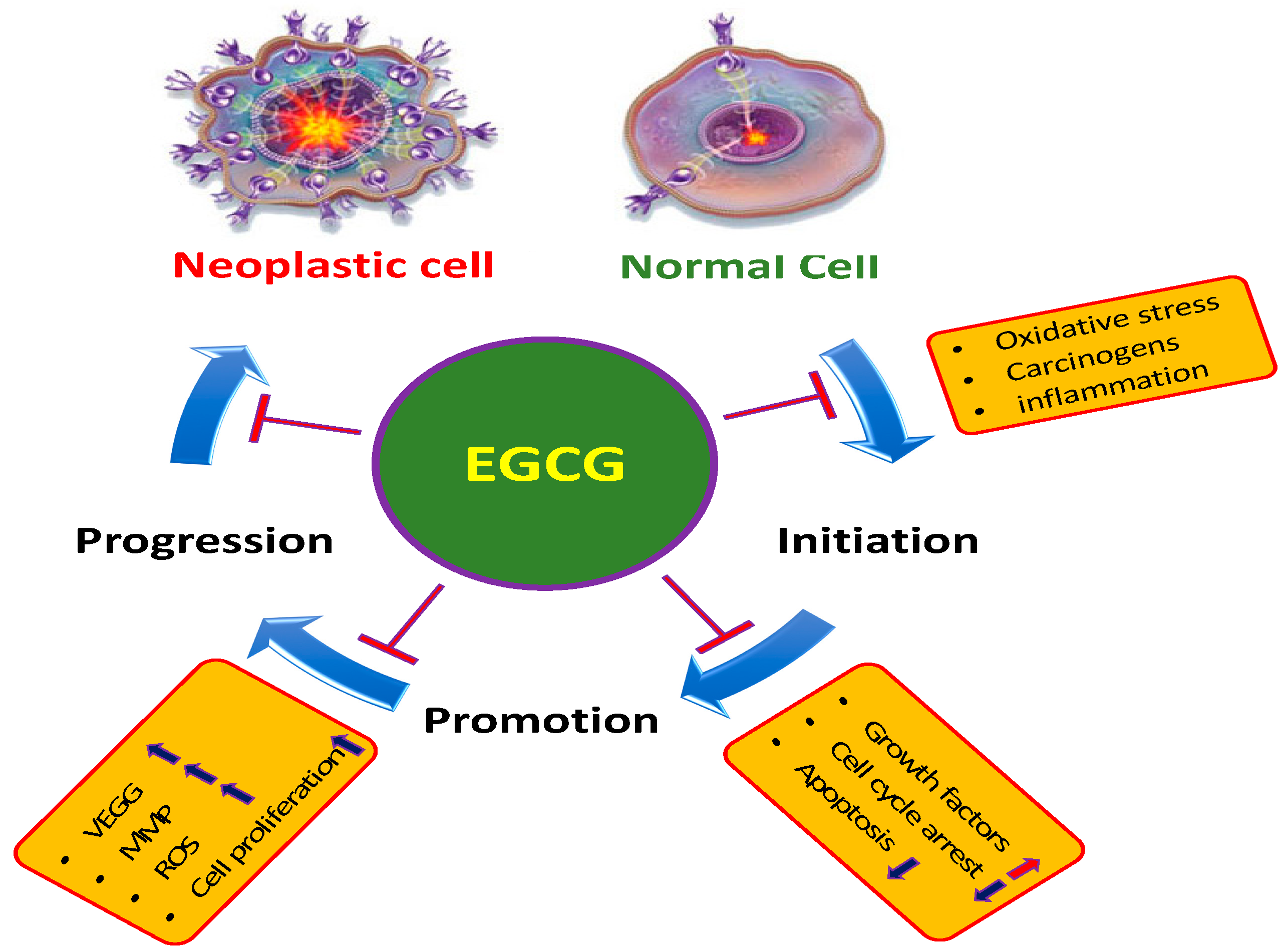This image is a detailed instructional drawing, likely from a textbook, that explains the stages of cell transformation. At the very top-left corner, there is a pictorial comparison of a neoplastic cell and a normal cell. The neoplastic cell label, written in red, illustrates a chaotic structure with a large red center and numerous purple protrusions. In contrast, the normal cell label, written in green, shows a more orderly structure with a smaller red center and slightly wavy edges.

Centrally positioned in the image is a green circle outlined in purple, containing the text "EGCG" in yellow. This circle acts as the hub of the cycle depicted in the diagram. Extending from the central circle are blue arrows that illustrate the progression of the cell transformation process, each marked with specific phases: initiation, promotion, and progression.

Starting from the normal cell, the diagram shows blue arrows labeled with relevant factors: from normal cell to initiation, labeled with "oxidative stress, carcinogens, inflammation"; from initiation to promotion, labeled with "growth factors increase, cell cycle arrest decrease, apoptosis decrease"; and from promotion to progression, labeled with "VEGG increase, MMP increase, ROS increase, cell proliferation increase." This cyclic process culminates back at the neoplastic cell, illustrating the transformation cycle resultant from different influences on cellular health.

Surrounding each phase labeling are yellow bullet points with red borders that emphasize key factors at each stage, designed to illustrate how various biological processes contribute to the development and transformation from normal cells to neoplastic cells, highlighting EGCG's role in this cycle.